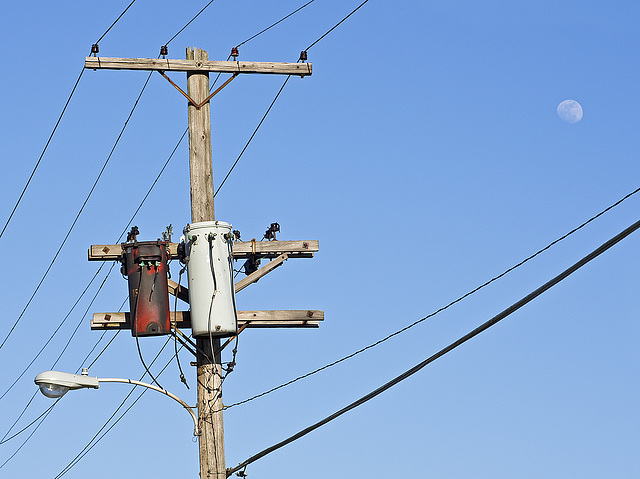This image captures a weathered wooden utility pole set against a sunny, cloudless blue sky. At the top of the pole, there is a T-shaped formation supporting four telephone wires. Attached to two horizontal wooden supports are two cylindrical objects: one larger, grayish-white canister and a smaller, reddish-black cylinder. Both canisters appear aged, with the red one showing signs of grease or corrosion, and each has three wires emerging from it. Further down the pole is a relatively new-looking streetlight. In the upper right corner of the sky, a nearly full white moon is faintly visible, adding a touch of serenity to the rugged scene.